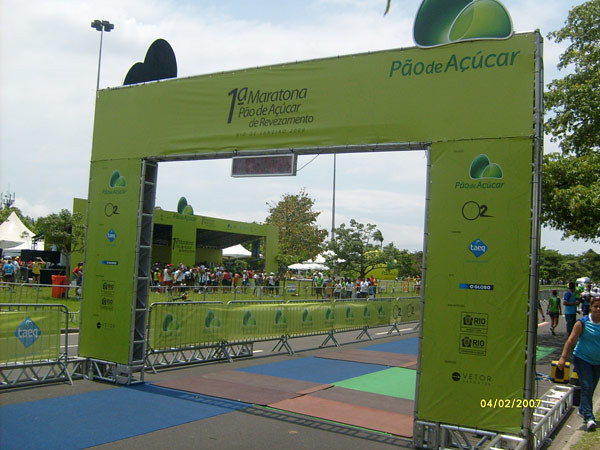The image captures a vibrant outdoor marathon finish line set on April 2nd, 2007. Central to the scene is a green portable archway adorned with dark green writing that reads "1A MARATONA PO O DE ACUCAR DE REVEZAMENTO," with a digital clock below it. Encircling this archway are numerous metal gates functioning as barriers, guiding the path for the runners. The track itself is a mosaic of colorful tiles, featuring blue, green, red, and dark brown hues, against a backdrop of lush green grass under a mostly cloudy sky with hints of blue. The attendees, gathered around the finish line, are dressed in various colored shirts, predominantly blue and green, evoking a lively and festive atmosphere. Stadium lights and surrounding trees enhance the setting, emphasizing the sunny and cheerful mood of the event. In the far distance, another green double archway is visible, and crowds of people are lined up along the fences, eagerly awaiting the marathoners.